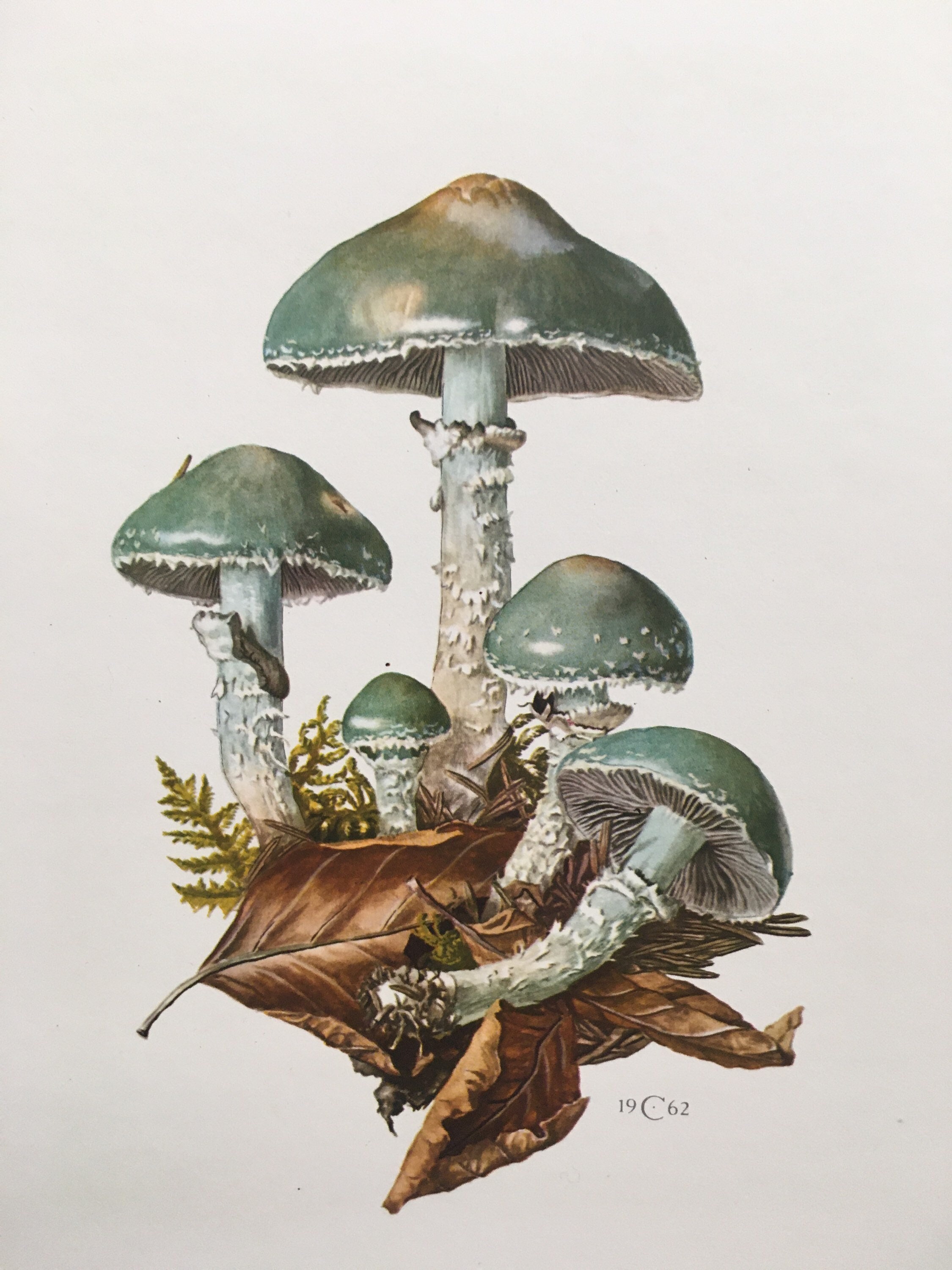In this detailed illustration set against a white background, five mushrooms of the same type, all featuring glossy green caps and white stalks, are depicted in various positions. The centerpiece of the image is the tallest mushroom, standing upright with a greenish-colored cap adorned with some growth along its sides. Flanking this central mushroom are two smaller ones on either side, positioned slightly underneath. Between these, a fourth, even smaller mushroom seems to have something looping around it, possibly resembling a frog or an unusual projection from the mushroom itself. The fifth mushroom lies on its side, appearing as if it has either been picked or has fallen over. Surrounding the fallen mushroom, you can see three crinkly, orange fall leaves, each with stems pointing in different directions—one towards the lower left corner, another towards the upper left corner, and the third hidden beneath the mushrooms. Additionally, there appear to be some brown leaves and fern leaves scattered near the bottom of the illustration. In the bottom right-hand corner, the marking "19C62" is visible, potentially indicating a date, a code, or a copyright mark.